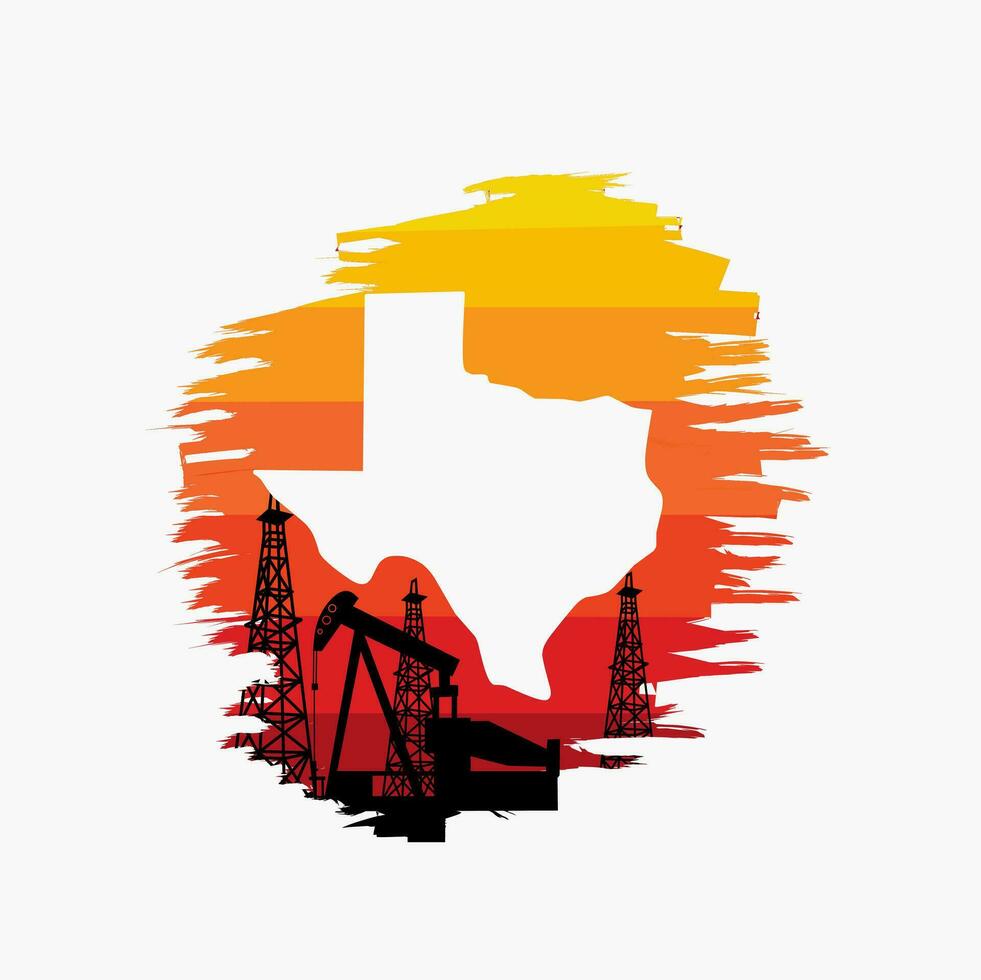The image showcases a striking graphic design of the state of Texas, set against a predominantly off-white background. At the center, there is a pure white silhouette of Texas, surrounded by a dynamic circular pattern composed of vibrant paintbrush lines. These lines radiate outward with sharp, flaring edges reminiscent of tassels, creating a sunset gradient transitioning from dark red at the bottom, through orange in the middle, to yellow at the top. Below this colorful display, the silhouette of an oil rig arm is prominently featured, accompanied by three tall, metal-framed oil towers, highlighting Texas's significance as an oil-producing state. This high-quality, visually appealing artwork would make an excellent design for a bumper sticker, t-shirt, or even the official Texas logo, with its bold, vibrant colors and detailed representation of the state's identity.